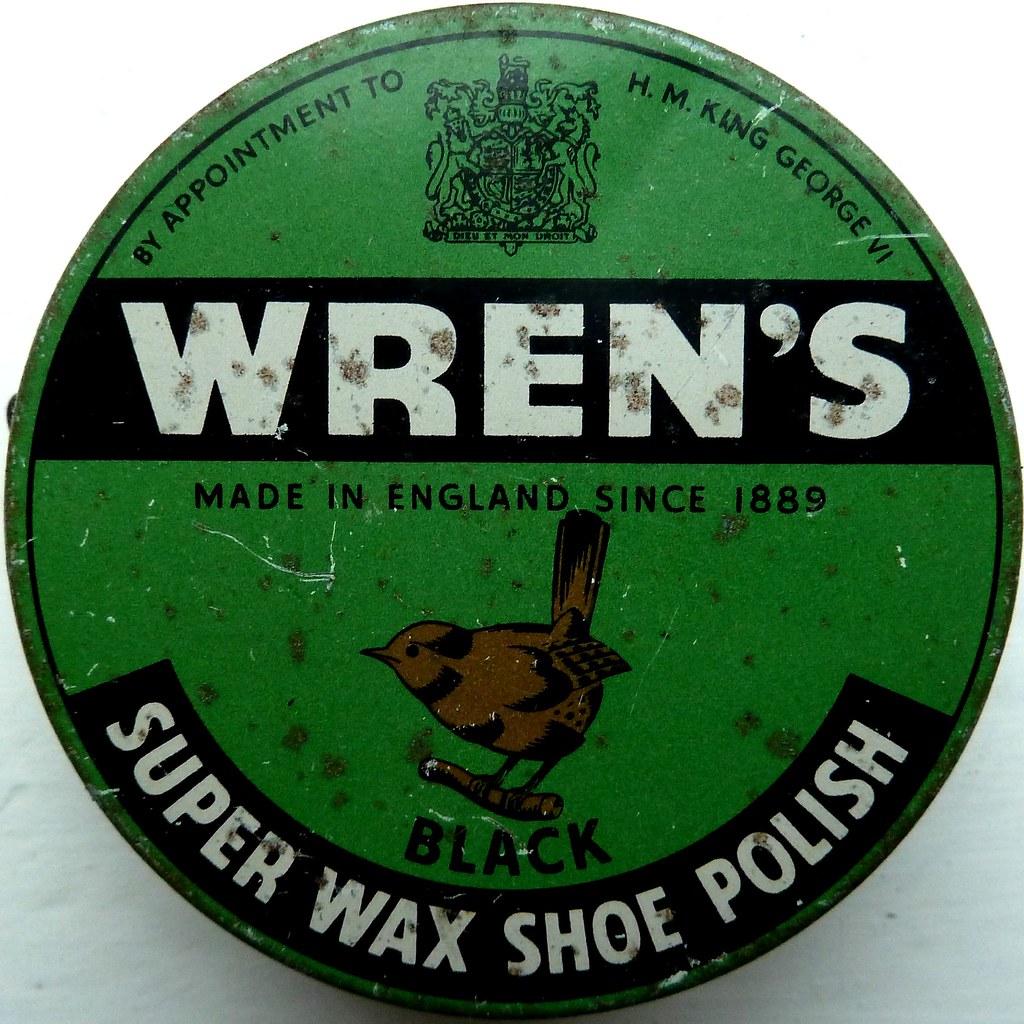This image showcases a worn, circular, bright green container lid with visible black spots indicative of wear and tear. The lid features a thin black ring around its perimeter. At the top of the circle, the text "By Appointment to H. M. King George VI" is written in black. Towards the upper center, a black banner with white letters spells out "WREN'S." Below this, it reads "Made in England Since 1889" in black font. The lid also includes an illustration of a brown bird perched on a small twig with the word "Super Wax Shoe Polish" displayed in a half-circular manner along the lower perimeter in a black banner with white letters.